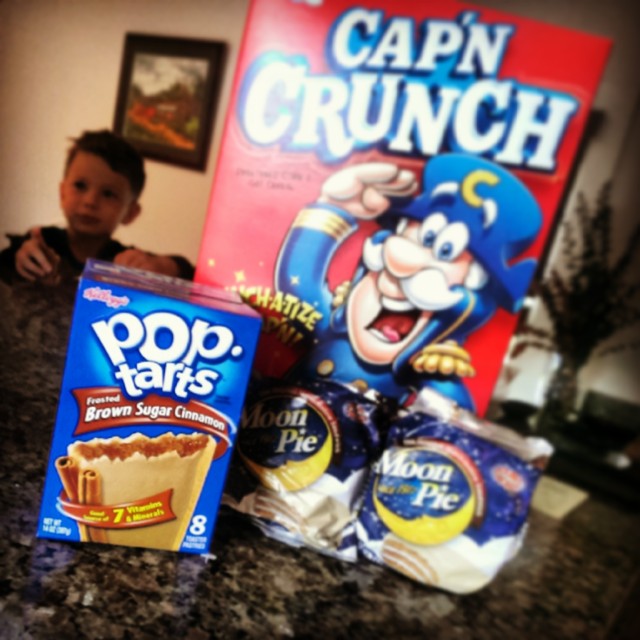A rustic brown counter table serves as the focal point, adorned with a quintessential breakfast spread. On the table, a large box of Captain Crunch breakfast cereal stands prominently, flanked to its left by a smaller box of Pop-Tarts in the classic brown sugar cinnamon flavor. In front of these two items, a package labeled Moon Pie completes the morning assortment. The background of the image is slightly faded, but a ghostly figure of a little boy, subtly visible on the left-hand side, suggests that this delightful breakfast awaits him. The morning light filtering into the scene further emphasizes the time of day, capturing not just a meal but a moment filled with nostalgic charm.